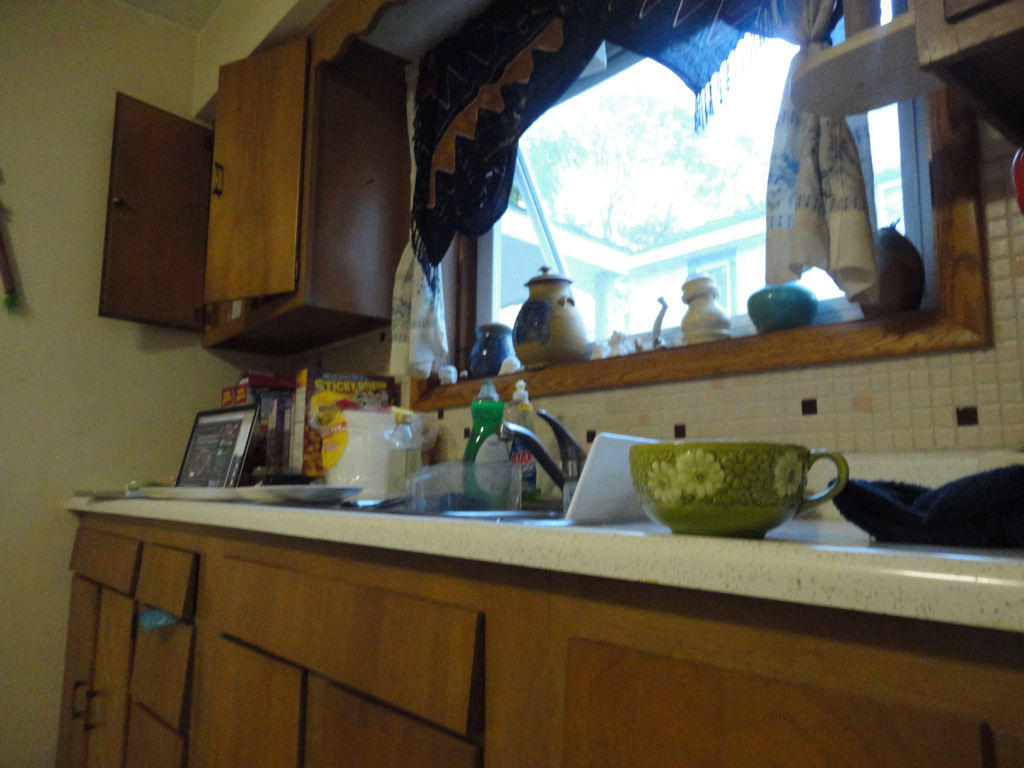The photograph captures a charming and nostalgic kitchen setting from a counter-level perspective, facing towards the sink. Above the sink, a window framed with blue tie-back curtains and a scarf valance allows natural light to pour in. 

Flanking the sink, the kitchen features vintage wooden cabinets with brassy handles and intricate carved wood detailing that add to the old-school charm. To the right of the sink, a homemade wooden paper towel holder is mounted on the side of the cabinet.

On the counter in front of the sink sits a green vintage coffee mug or teacup. Inside the sink, on the right side of the basin, a white plastic cutting board leans conspicuously. The back ledge of the sink hosts a green bottle and a yellow bottle of liquid dish soap, standing side by side.

Under the far left cabinet, cookbooks and cereal boxes are neatly lined up on the counter. At the very end of the counter on the left-hand side, near the wall, an open laptop hints at modernity amidst the vintage setting.

The windowsill above the sink is decorated with several handmade ceramic pots with lids—one blue and another of stoneware with blue trim and design. Additionally, a visible turn handle indicates the window is tilted open from top to bottom. Scattered across the windowsill are various other objects, their details obscured from view.

The backsplash consists of small white tiles sprinkled with occasional black and pink tiles, providing a quaint and cozy backdrop to this homey kitchen scene.